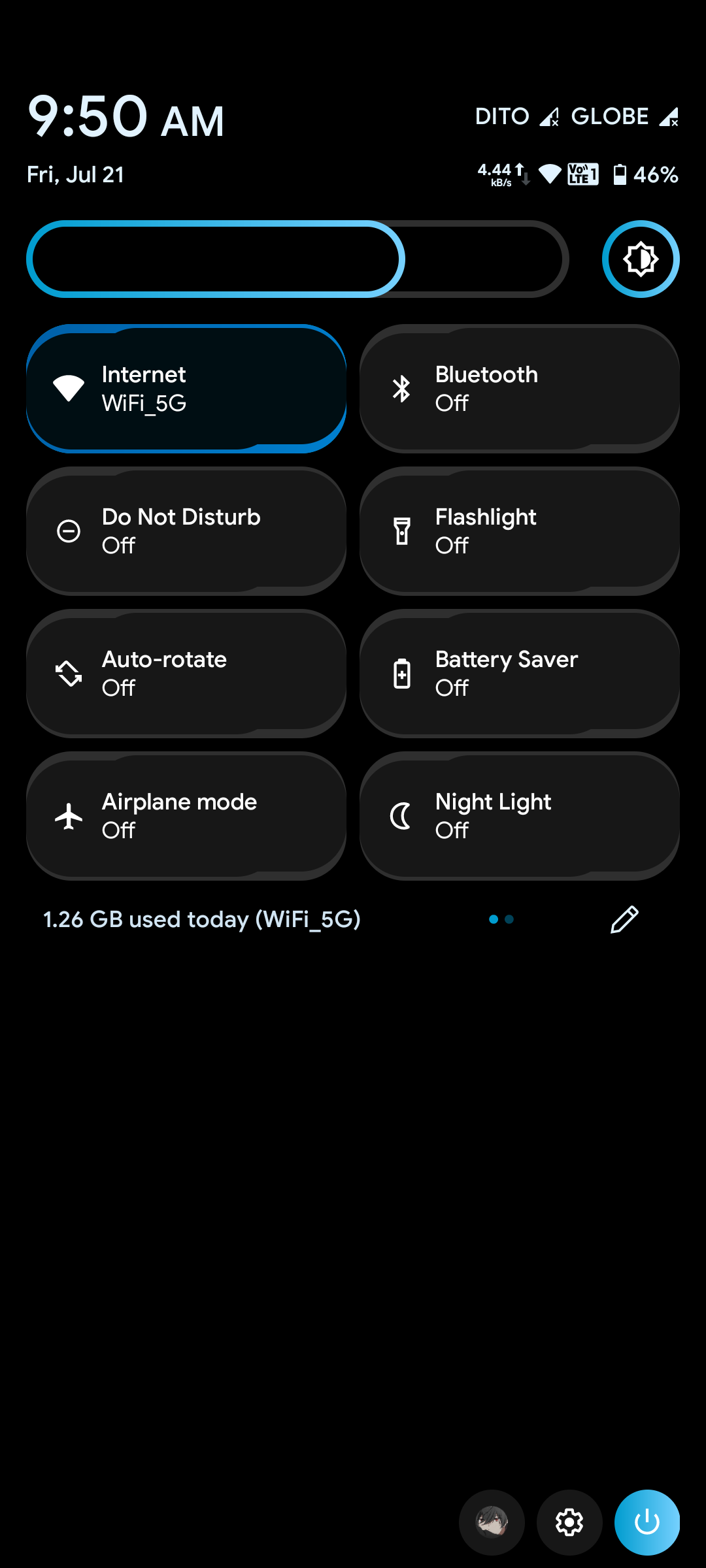The image depicts a smartphone screen displaying the status bar and Quick Settings menu. The background is entirely black, and at the top of the screen, the time is shown as 9:50 a.m. alongside the date, Friday, July 21st. The battery icon on the left indicates a 46% charge. Additionally, other small icons are present at the top of the screen.

Beneath the status bar, there's a text input area outlined by a teal, shiny border, currently empty. Below this, various options in the Quick Settings menu are displayed. The Wi-Fi network is connected to "Wi-Fi_5G," and Bluetooth is turned off. Other settings such as 'Do Not Disturb,' 'Flashlight,' 'Auto-Rotate,' 'Battery Saver,' 'Airplane Mode,' and 'Night Light' are all shown as off.

At the bottom of the screen, data usage information indicates "1.26 GB used today" and reiterates the Wi-Fi connection to "Wi-Fi_5G." Two blue dots and the outline of a pencil icon are also visible.